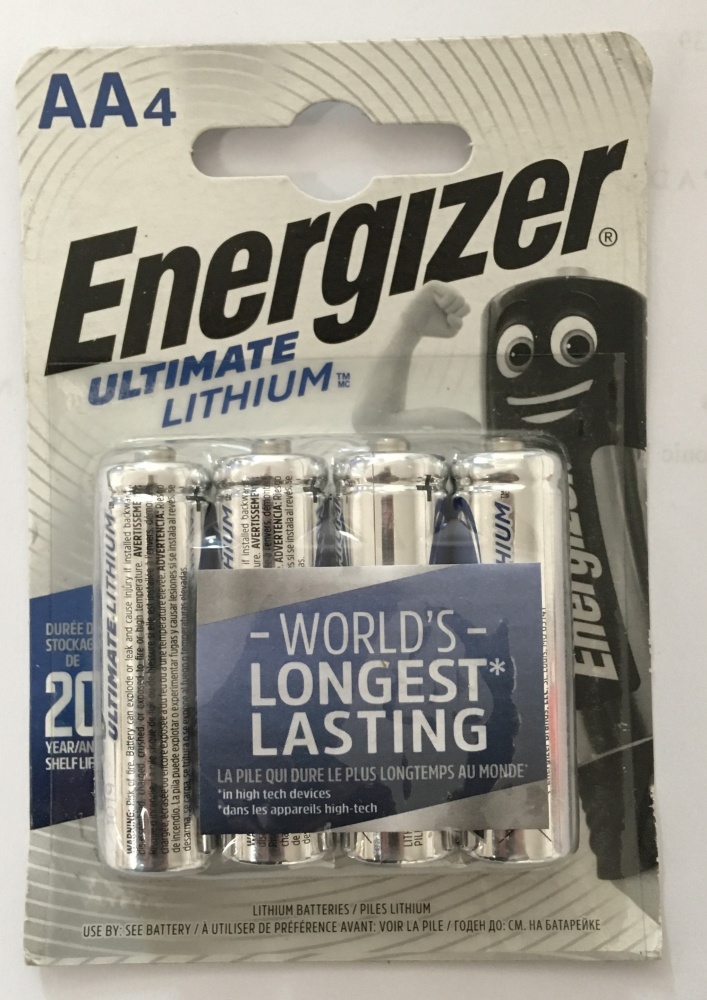This image depicts the back packaging of Energizer Lithium AA batteries. The cardboard backing features a white background with a circular silver pattern. At the top of the packaging, there's a small alcove designed for hanging the product on a store peg. Directly below this hanging section, the Energizer and SanDisk logos are prominently displayed on the left, while smaller corporate symbols are situated on the top right. The text "Ultimate" is written in gold and blue, and just below in blue text, it reads "Lithium™". This text is partially covered by the plastic housing that encases the batteries.

The packaging contains four shiny silver AA batteries, arranged with their positive terminals pointing slightly to the right. Above the batteries, there's an insert that claims "World's Longest Lasting Electronics," written in white text. There is also some small, detailed subtext along the background and at the bottom of the cardboard cutout. On the right side of the packaging, a cartoon features an Energizer battery personified with a muscular human arm.